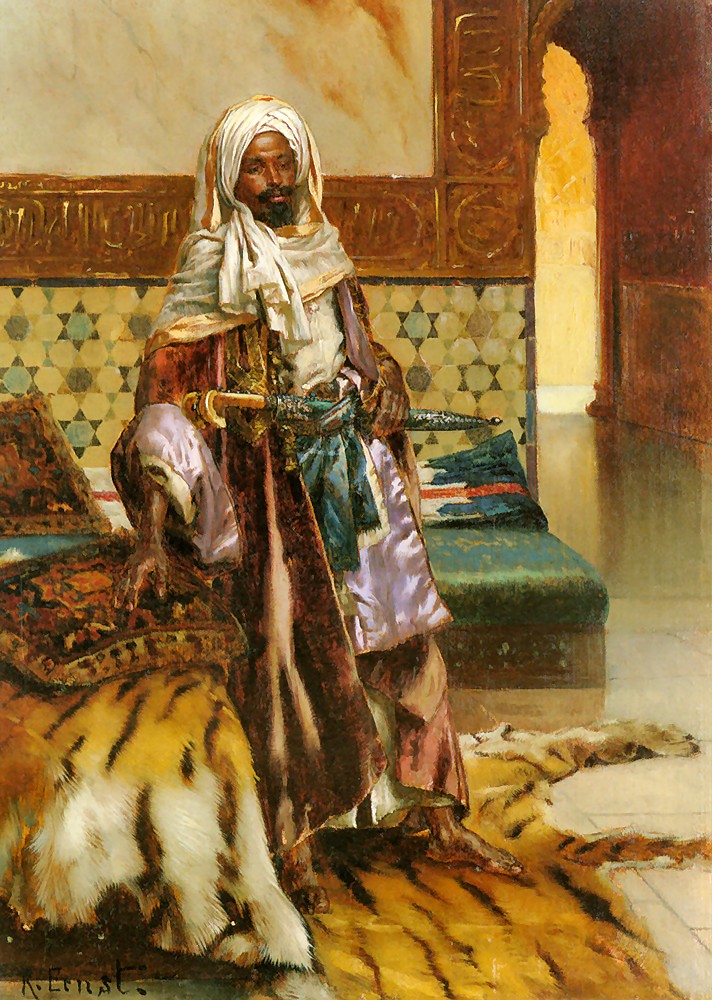This detailed orientalist painting portrays a dark-skinned man standing barefoot on a luxurious tiger-skin rug. His attire is opulent: he wears a long, richly colored robe in shades of pink, red, and white, complemented by a blue belt or shawl. Draped over his head is a white turban, and he sports a beard or goatee with a mustache. In his right hand, he rests on a pillow atop the tiger rug, while holding what appears to be an umbrella with a blue top and a golden yellow handle. He stands next to a bed adorned with similarly luxurious tiger-skin and richly embroidered golden brown pillows. Behind him, there is another piece of furniture—it could either be a couch or another bed—situated against a backdrop that includes a detailed view of the tiled floor leading into a hallway and the intricately decorated walls of the room. The artist's signature, "K. Ernst," is visible in the lower left corner, marking this scene of Middle Eastern interior décor complete with opulent textiles and furnishings.